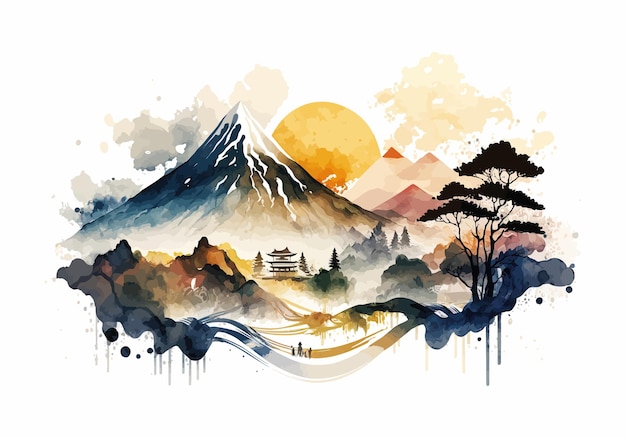The image depicts a beautifully detailed painting inspired by Asian culture. At its center is a towering, sharp-pointed mountain with snow-capped peaks, painted with shades of gray, black, and brown. The scene is bathed in the warm glow of a large, bright orange sun, either setting or rising behind the mountain, casting a serene light over the landscape. Surrounding the mountain, there are clouds painted in hues of pink, gray, and white, with fog rolling in, adding to the mystical atmosphere.

To the left of the mountain lies some sparse shrubbery, while the right-hand side features several tall evergreen trees standing prominently against a backdrop of smaller mountain peaks tinged in pink. Nestled at the base of the mountain, there's a small shrine or Japanese house, subtly suggesting human presence and traditional architecture. In the valley below, a family of four can be seen walking toward their home, adding a touch of warmth and life to the serene, natural setting.

The foreground is painted with a mix of green foliage and blue tones, depicting the land and trees in varied shades of brown, gray, and green. This harmonious blend of colors and detailed elements creates a tranquil and picturesque mountain scene, capturing the essence of nature’s beauty with artistic finesse.